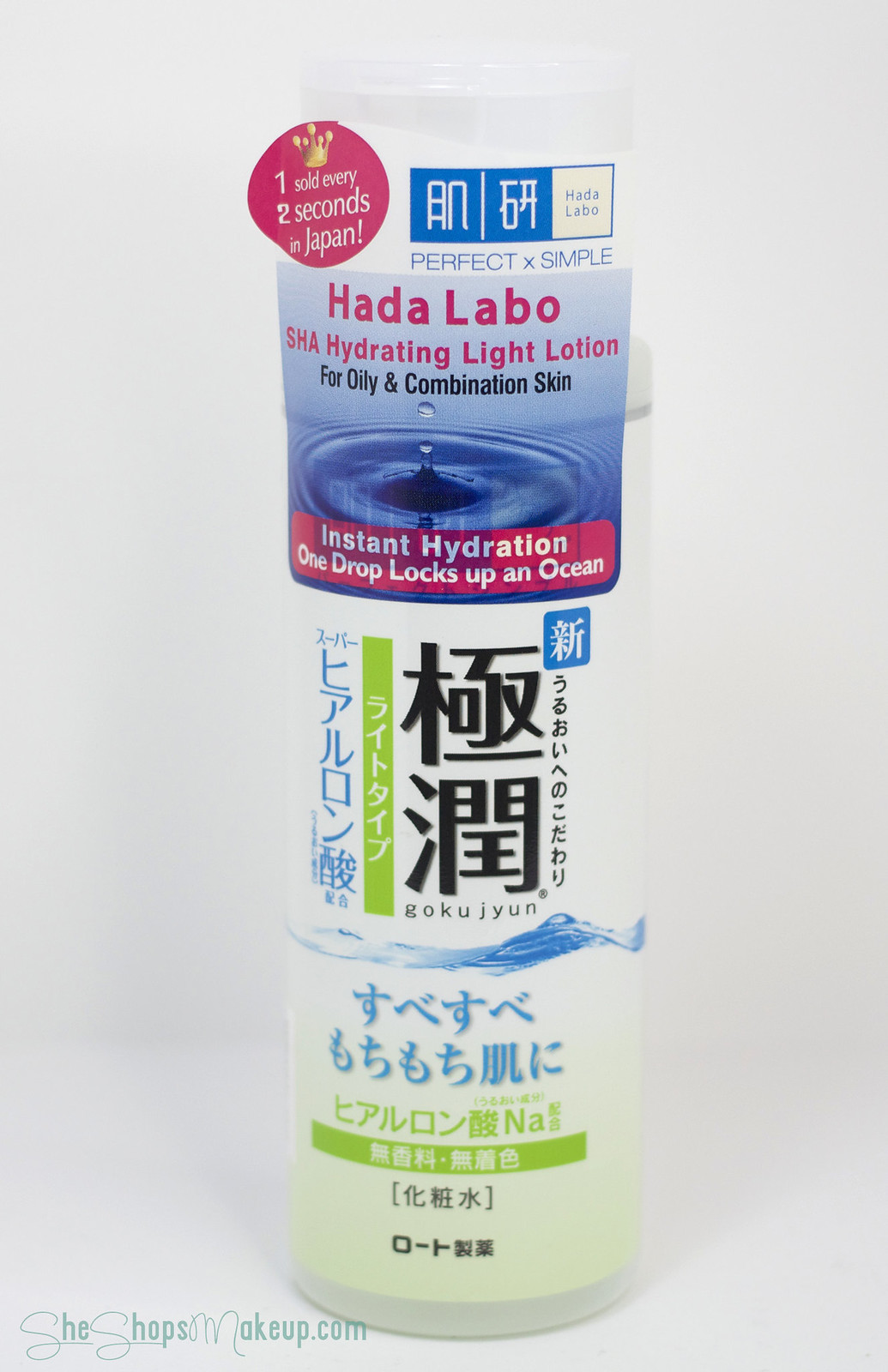This image showcases a Japanese product, specifically the Hada Labo SHA Hydrating Light Lotion for oily and combination skin. The product is presented in a clear cylindrical tube with a white-to-light-green ombré lotion visible inside. At the top-left of the bottle, there is a prominent pink circle with a crown that claims "One sold every two seconds in Japan" and emphasizes its popularity. Below this, the product promises "Instant Hydration: One drop locks up an ocean," highlighting its hydrating properties. The packaging features a picture of a water droplet splashing into water, reinforcing its moisture-rich benefits. The text is primarily in Japanese, with some English phrases, making the branding accessible to a diverse audience. Additional text at the bottom of the image includes the potential volume of the product, possibly indicated by "O dash" which could mean four ounces, and a web address "keyhopsokep.com".